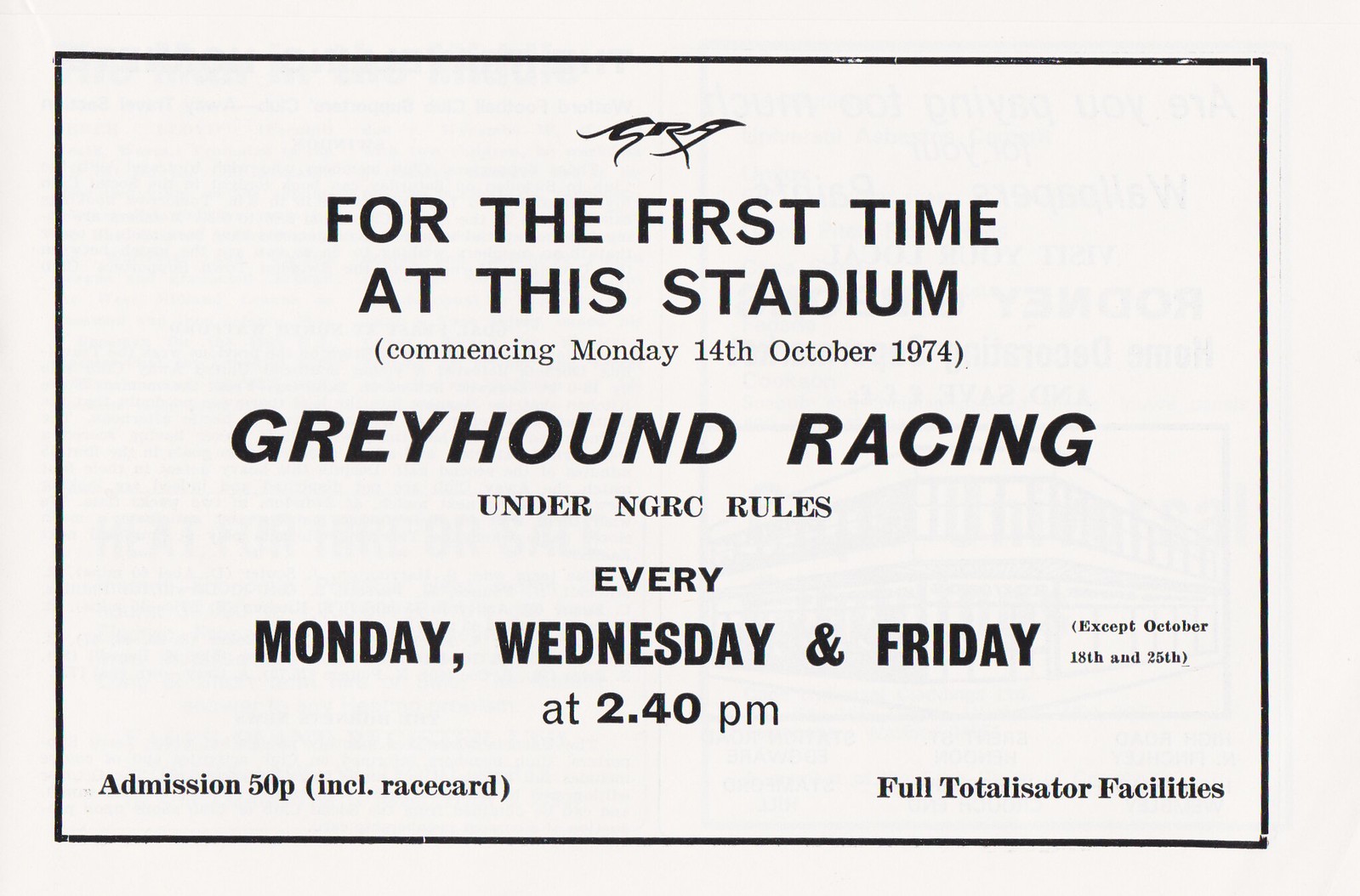This monochromatic newspaper advertisement, set against a white background with a thin black border, announces the commencement of Greyhound Racing for the first time at this stadium. The text is prominently displayed in black, with a cursive, somewhat diagonal style forming the headline. At the top, it reads, "For the first time at this stadium," with "commencing Monday, 14th October 1974" in smaller letters beneath it. Below, in larger text, it proudly declares "Greyhound Racing under NGRC rules every Monday, Wednesday, and Friday" with a note to the right stating "except October 18th and 25th." The announcement continues with the racing time "at 2.40 p.m." In the bottom left corner, it states, "admission, 50p, including race card," while the bottom right corner mentions "full totalizator facilities." This detailed layout aims to attract enthusiasts to this new, thrice-weekly event.